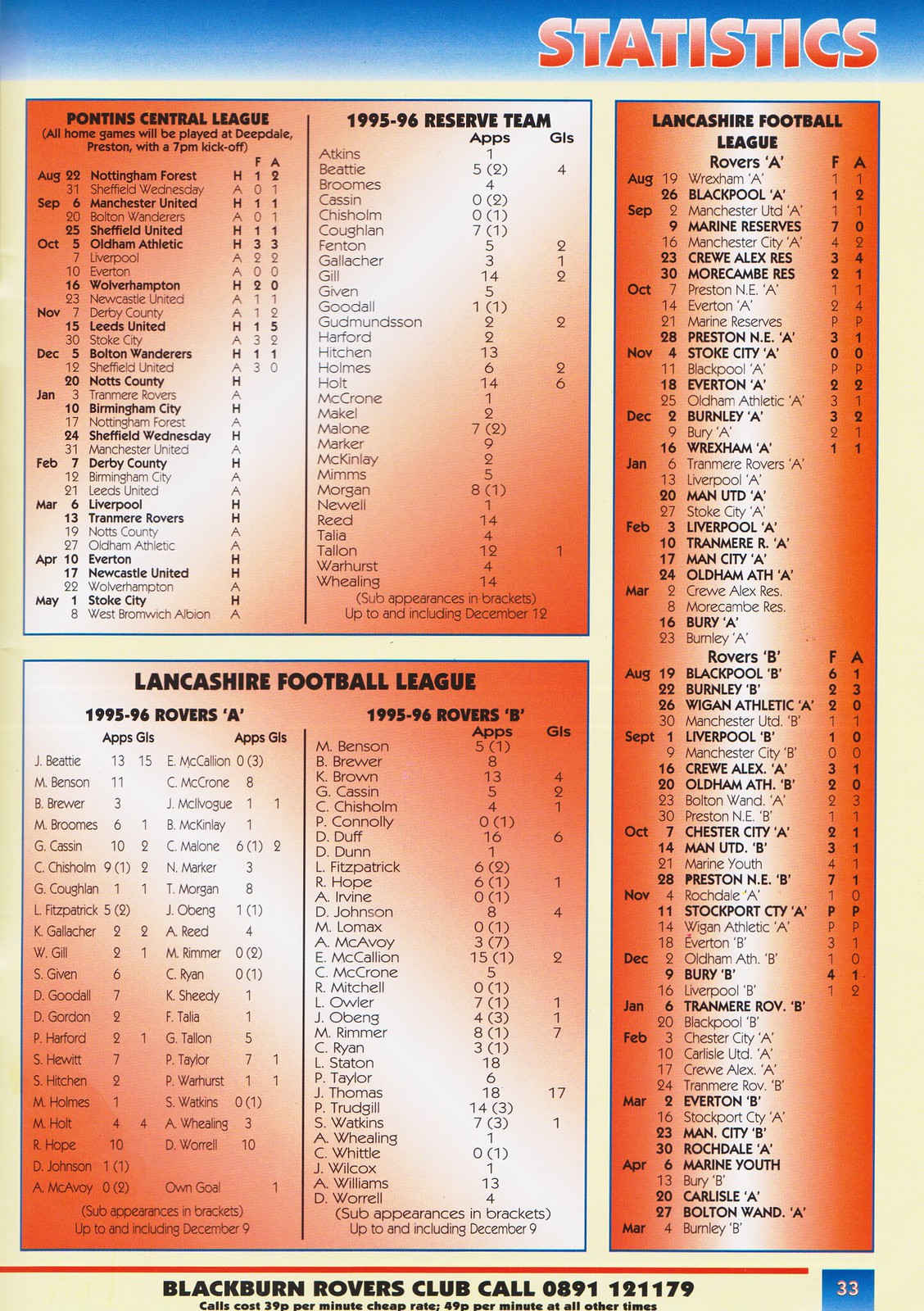The image showcases a detailed statistic sheet from a football league, prominently featuring the Blackburn Rovers Football Club. The sheet includes team statistics and game details, displayed on a card, reflecting the school's blue and orange colors. It highlights games played in the Ponton Central League, with all home matches held at Deep Dale Preston, starting at 7 p.m. The chart tracks scores from August 22nd to December 12th, listing matchups against prominent teams like Nottingham Forest, Manchester United, Sheffield United, Oldham Athletic, Wolverton, Wolverhampton, Leeds United, and Bolton Wanderers. Additionally, it features the 1995 to 96 reserve team players' roster, with names such as Atkins, Kaysen, Given, Hartford, Mims, Morgan, Talia, and Wheeling. The document also provides details on the Lancashire Football League 1995 to 96 for Rovers A and B teams, including sub appearances noted up to December 9th. At the bottom, it mentions the Blackburn Rovers club contact number and call costs, emphasizing the comprehensive nature of the club's season statistics.